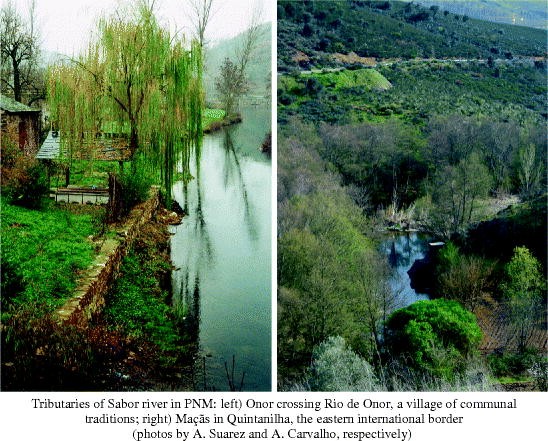The image features two vibrant, saturated color photographs of river tributaries, with the left showcasing a scene titled "Tributaries of Sabor River in PNM," attributed to A. Suarez. This photo captures a serene tableau with a small stone building alongside the riverbank, bordered by bright green grass and a prominent willow tree at the center. Surrounding the pond or small lake, leafless trees are reflected in the calm water, set against a backdrop of gentle hills. The right photograph, taken by A. Cavarjo, is labeled "Honor Crossing, Rio de Honor, a village of communal traditions, right," and "Macas in Quintanilla, the eastern international border." It displays a more mountainous and green terrain, dominated by lush vegetation, trees, and bushes around a swampy area. Here the landscape is characterized by a flat field dotted with dark green bushes, creating a picturesque scene that mirrors communal rural life despite being at an international border. Both images collectively emphasize the natural beauty and tranquil essence of these regions, unified by their deep green hues, blue waters, and overall pastoral charm.